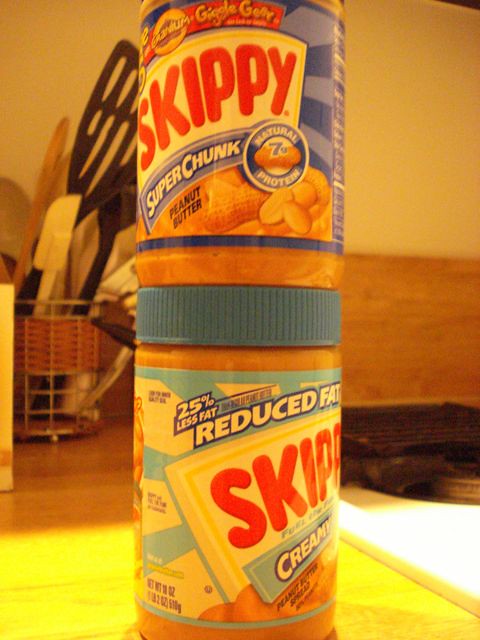In this indoor color photograph, we see a detailed and slightly dimly lit kitchen scene with two brand-new, unopened Skippy peanut butter jars prominently stacked atop a wooden countertop. The image, which has a yellowish tint and a slightly grainy quality, is framed in a portrait orientation, being roughly 50% taller than it is wide.

The bottom jar features a light blue lid and a label indicating "Skippy" in red letters, along with "25% Less Fat" and "Reduced Fat" in white letters. The label is turned slightly to the right, hiding some text, but we can discern it is creamy peanut butter.

The top jar, slightly cut off at the top, features a dark blue lid with a label that reads "Skippy Super Chunk" and "Natural, 7 grams of protein." The label also displays images of peanuts both in and out of their shells.

In the background, to the left, there is a metal container holding cooking strainers and spatulas, partially obscured by a woven basket with thin vines. The background further reveals a light tan wall in the upper corners. To the right, there's an indistinct black item on the table, contributing to the dim and cozy kitchen atmosphere.